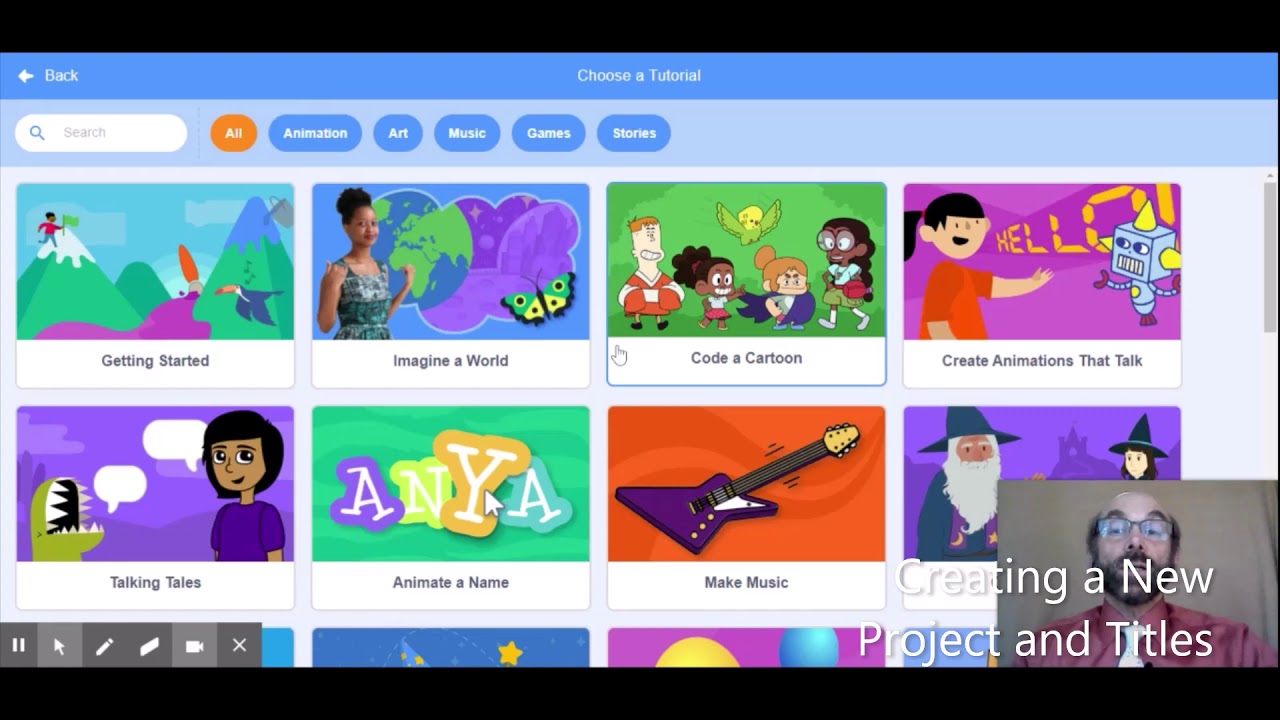This image appears to be a screenshot taken on either a tablet or a computer screen. It is framed with black banners at the very top and bottom. The primary focus is a user interface with a light blue banner stretching horizontally across the top. In the upper left corner, a white arrow pointing left is accompanied by the word “Back” in white font. Centered within this banner, it reads, “Choose a Tutorial" in white text.

Beneath the “Back” button, a white, cylindrical search box contains a diagonal magnifying glass icon and the word “Search.” Adjacent to it is an orange cylindrical button labeled “All” in white text. Following this orange button is a series of category buttons with a blue background, displaying the options: “Animation,” “Art,” “Music,” “Games,” and “Stories.”

Below this row of options, eight distinct tutorial boxes are arranged:

1. **Getting Started**: This box features an illustration of a person ascending a mountain.
2. **Imagine a World**: Depicted is an African descent woman pointing towards a multicolored butterfly against a globe backdrop.
3. **Code a Cartoon**: Showcases four cartoon characters of diverse ethnicities with a bird perched above them, all highlighted in blue.
4. **Create Animations that Talk**: Presents an image of a girl saying “Hello” to a robot.
5. **Talking Tales**: Features a likely Indian descent girl speaking, with narrative bubbles leading to an open-mouthed dinosaur.
6. **Animate a Name**: Illustrates the name “Anya” in various colors.
7. **Make Music**: Displays an electric guitar.
8. **Creating a New Project and Titles**: Shows a Caucasian man with glasses, a full beard, and bald top, dressed in a red button-up shirt over a white shirt or possibly a tie.

This detailed layout offers a user-friendly visual guide to select from various tutorials.